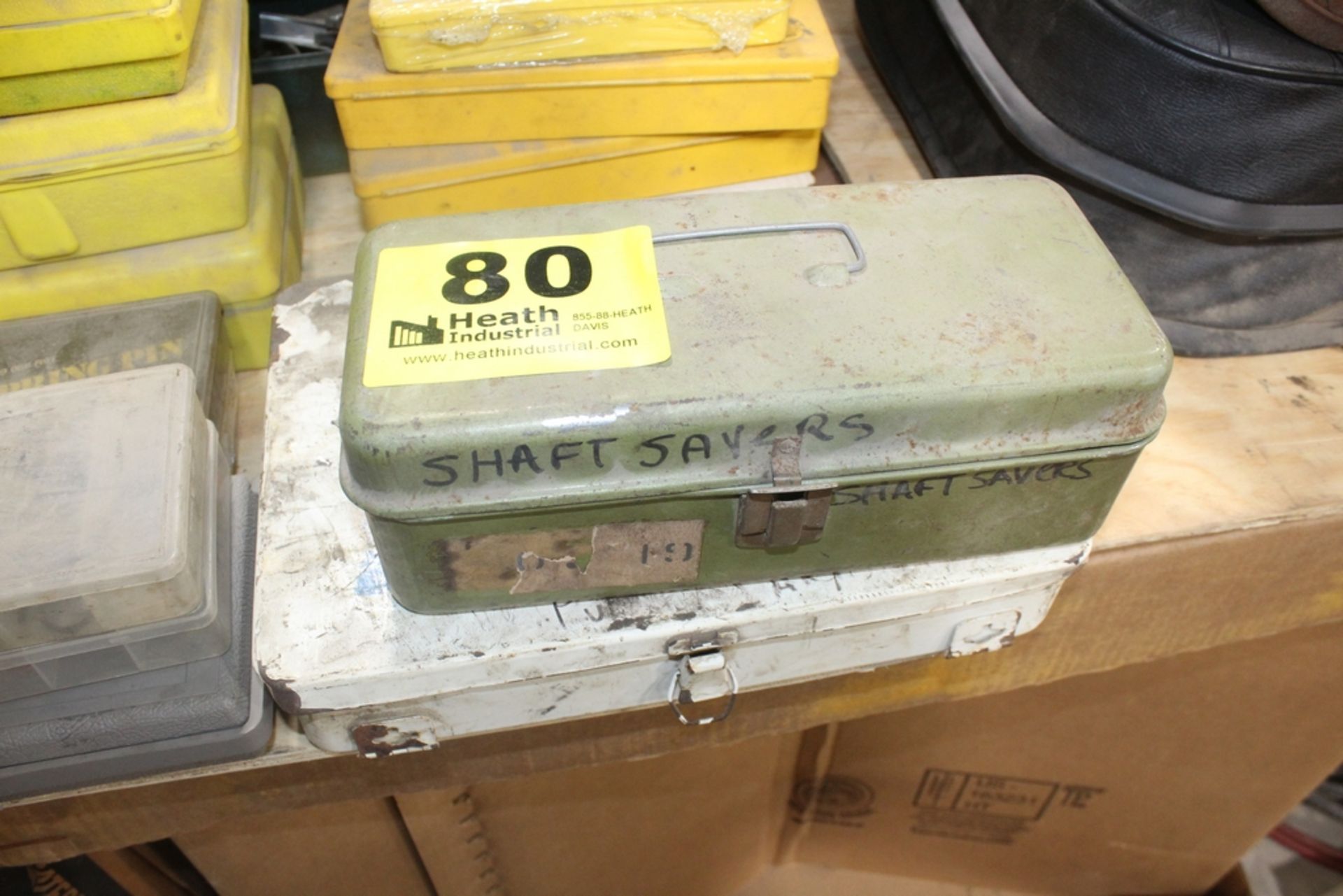In this photograph, a collection of various toolboxes and plastic containers are meticulously stacked on a wooden counter made of unpolished wood. At the bottom of the stack lies a heavily scraped, flat rectangular white box adorned with visible brown and gray marks and slight rust, secured by clasps in the front. Resting atop it is a green metal toolbox, which has the words "Shaft Savers" both hand-written in black marker on its lid and printed on its body. A large yellow sticker bearing "AD Health Industrial" is prominently displayed on the lid. Above these, scattered and stacked, are containers of different colors, including transparent and yellow ones. In the upper right corner of the image, part of a black case is visible, possibly the corner of a cloth suitcase. The setting appears to be a workshop or garage, a utilitarian space where tools and supplies are stored and organized. The overall scene suggests a well-used and practical area dedicated to maintenance or craftwork.